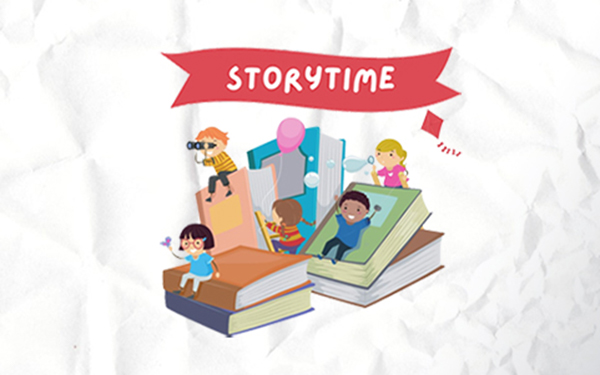This vibrant, cartoon-styled advertisement is set against a white background designed to look like crumpled paper. Dominating the top of the image is a bold red banner with white lettering that reads "Story Time." The scene below the banner showcases a playful and imaginative depiction aimed at promoting reading among children.

In the foreground, there are several sets of oversized books arranged in varied positions: some are lying flat while others stand upright, forming makeshift playground structures. Five animated children, each portrayed with distinct features, are engaging with the books in different ways. One child with short hair uses an angled book as a slide, gliding down with joy. Another sits atop a stack of books, while elsewhere, a girl is blowing bubbles. There’s a pink balloon floating nearby and a red kite soaring in the background, its tail trailing whimsically. In the midst of the fun, a ginger-haired boy peers through binoculars, adding a touch of adventure to the scene. 

Additionally, the image includes a girl drawing on an easel, symbolizing the creativity and exploration that come with reading. This graphic effectively conveys that storytime can unlock new worlds and adventures, making books a source of fun and imagination.

Overall, the image promotes the idea that reading is an exciting and enjoyable activity, potentially suggesting that it could be featured in a library or another venue dedicated to children's literacy.